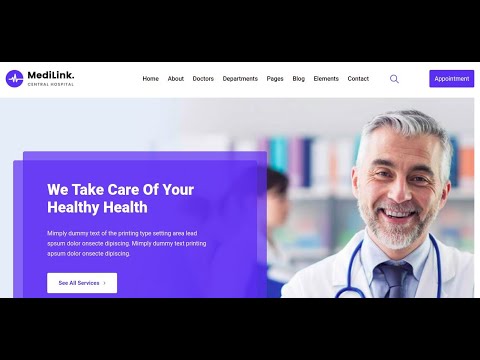The image depicts a left-to-right horizontal screenshot of a website, viewable on a smartphone or computer. The background is a solid jet black strip running across the top and bottom of the screen, providing a striking contrast to the main content. Overlaying this black backdrop is a prominent white box. 

Located on the left-hand side of the white box is a small purple circle displaying the text "MediLink, Central Hospital." Adjacent to this is a navigation menu with black text containing options such as Home, About, Doctors, Departments, Pages, Blog, Elements, and Contact, accompanied by a magnifying glass icon for search functionality. A noticeable purple button with white text labeled "Appointment" is also placed next to this menu, ready for user interaction.

The main image within the box features a doctor in a lab coat with a stethoscope draped around their neck. The background of the image is slightly blurred, showing indistinct bookshelves and a woman, enhancing the focus on the doctor. 

Additionally, the image contains several purple overlay boxes. One declares, "We Take Care of Your Healthy Health," followed by a brief explanatory blurb. Below this, there is a white rectangular box with purple text reading "See All Services," which appears clickable.